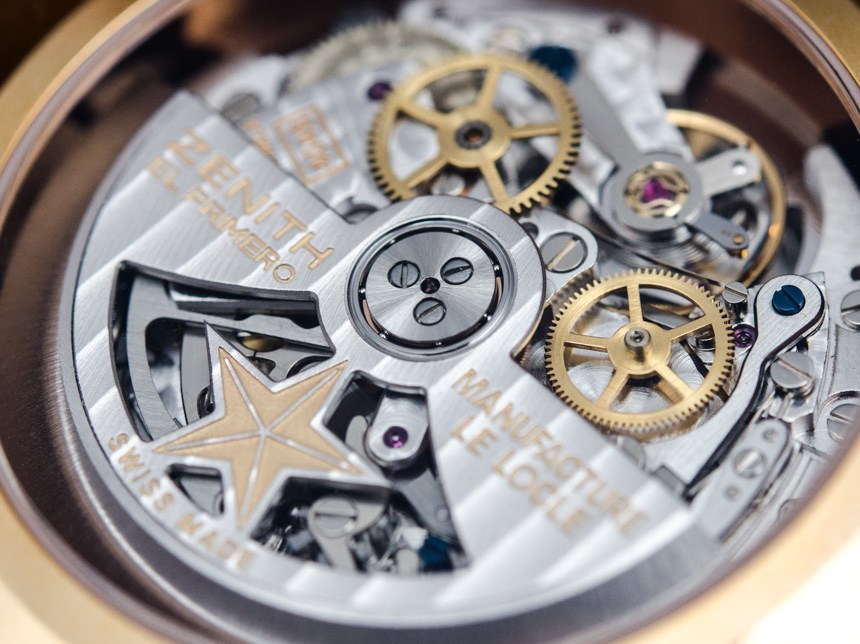The image provides a detailed, close-up view of the intricate inner workings of a Swiss-made watch, likely a Zenith El Primero model. Dominating the composition are the precise, well-crafted gears and mechanisms, primarily rendered in shimmering silver metalwork. At the top, two prominent gold gears stand out amidst the machinery. Below, the brand name "Zenith El Primero" is elegantly inscribed in gold lettering, matching the hue of the gears. Adjacent to it on the right, additional gold-scripted text reads "Manufacture Le Locle," accompanied by a matching gold star, with "Swiss Made" inscribed just beneath. Notably, a purple jewel or gem is situated near the gears, adding a touch of color to the otherwise metallic palette. The overall impression is one of meticulous craftsmanship and timeless precision, characteristic of Swiss horology.